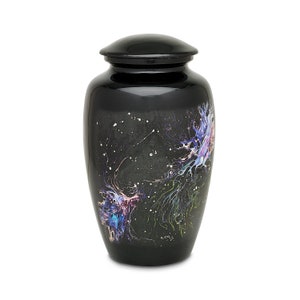The image features a small black urn, measuring approximately two to three inches in height. The urn has an oval shape with a perfectly fitting, somewhat shiny black lid. The exterior showcases a space-inspired design adorned with a vibrant mix of pink, blue, and purple hues, along with scattered white dots resembling stars. The celestial theme is further emphasized by depictions of constellations and galaxies, giving the urn a galactic or space-age aesthetic. The intricate design contrasts starkly against the black background, creating an impression of the night sky. The context of the image is focused solely on the urn, with no additional background elements visible.